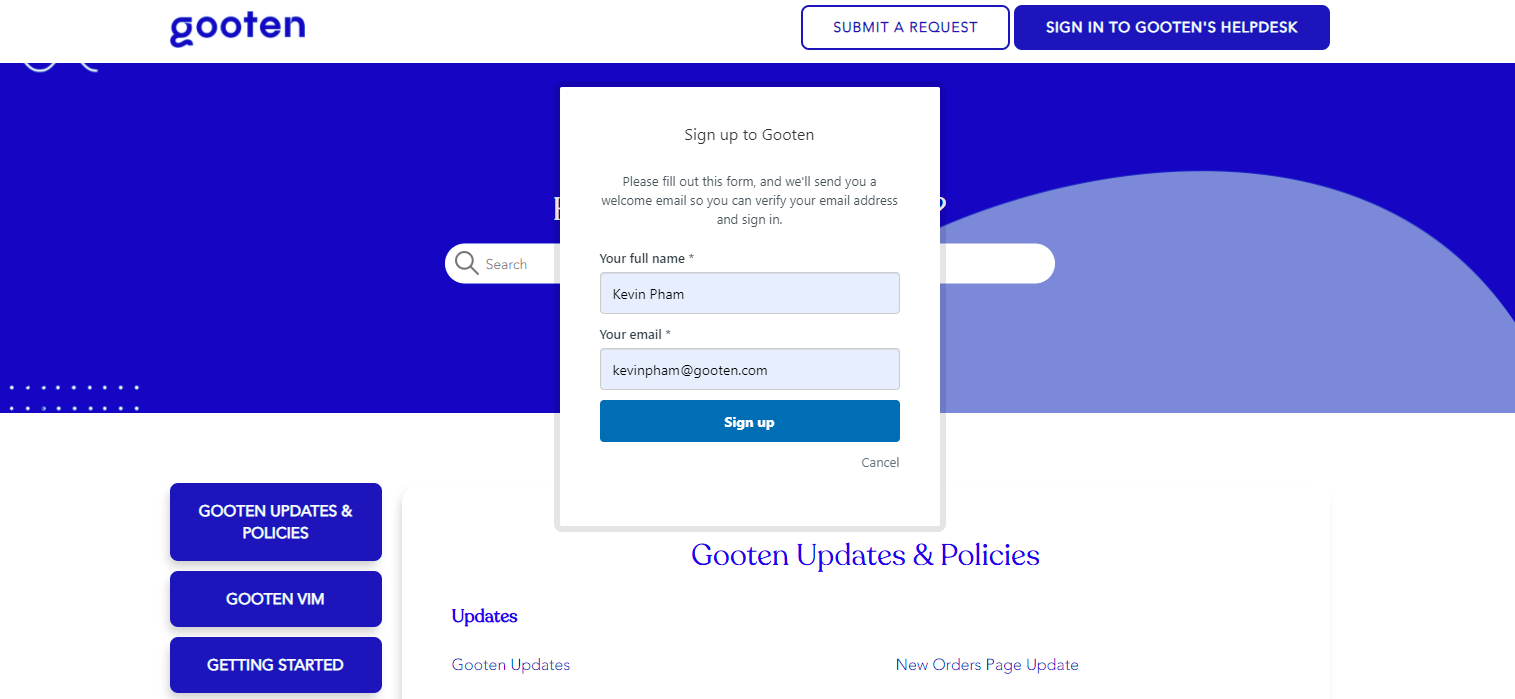The screenshot showcases the main page of Gooten's website. In the top left corner, the company's name, "Gooten," is prominently displayed. Various action buttons are visible, including options to "Submit a Request," "Sign into Gooten's Help Desk," and "Sign Up to Gooten." Fields to input "Your Full Name" and "Your Email" are provided, along with buttons for "Sign Up" and "Cancel." 

The page also features links to "Gooten Updates and Policies," "New Gooten," and "Gooten VIM," with a section dedicated to "Getting Started" with Gooten. The background of the page is a soothing shade of blue, and a search bar is subtly placed in the background. Notably, "Gooten" is meticulously spelled out as "G-O-O-T-E-N" multiple times for clarity.